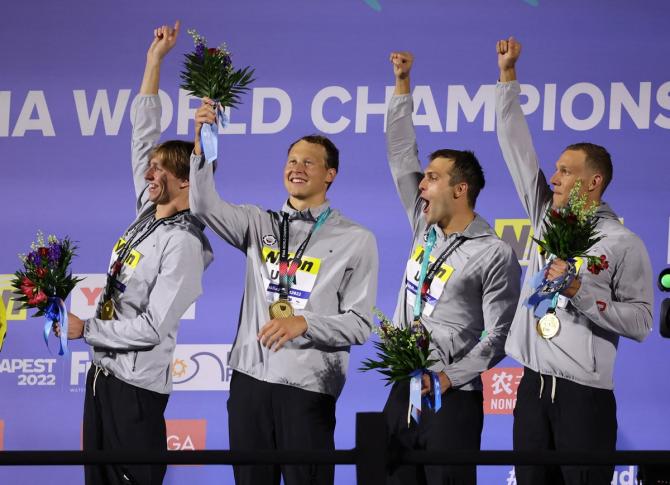In this modern photograph, we see a jubilant team of four young white male athletes, possibly Olympians, celebrating their recent victory. They stand atop a podium, each adorned in matching grey jackets with the Nikon USA logo prominently displayed on their chests and black pants, signifying their team unity. Around their necks hang medals, likely gold or bronze, signifying their achievement. Each member triumphantly raises his right hand, mouths open in cheerful exclamation, while clutching a bouquet of flowers in their left. The backdrop features a large blue panel emblazoned with "World Championships" in white lettering, alongside numerous sponsor logos, hinting at a prestigious event, possibly from the year 2022. Their radiant smiles and the celebratory atmosphere capture a moment of shared triumph and pride.